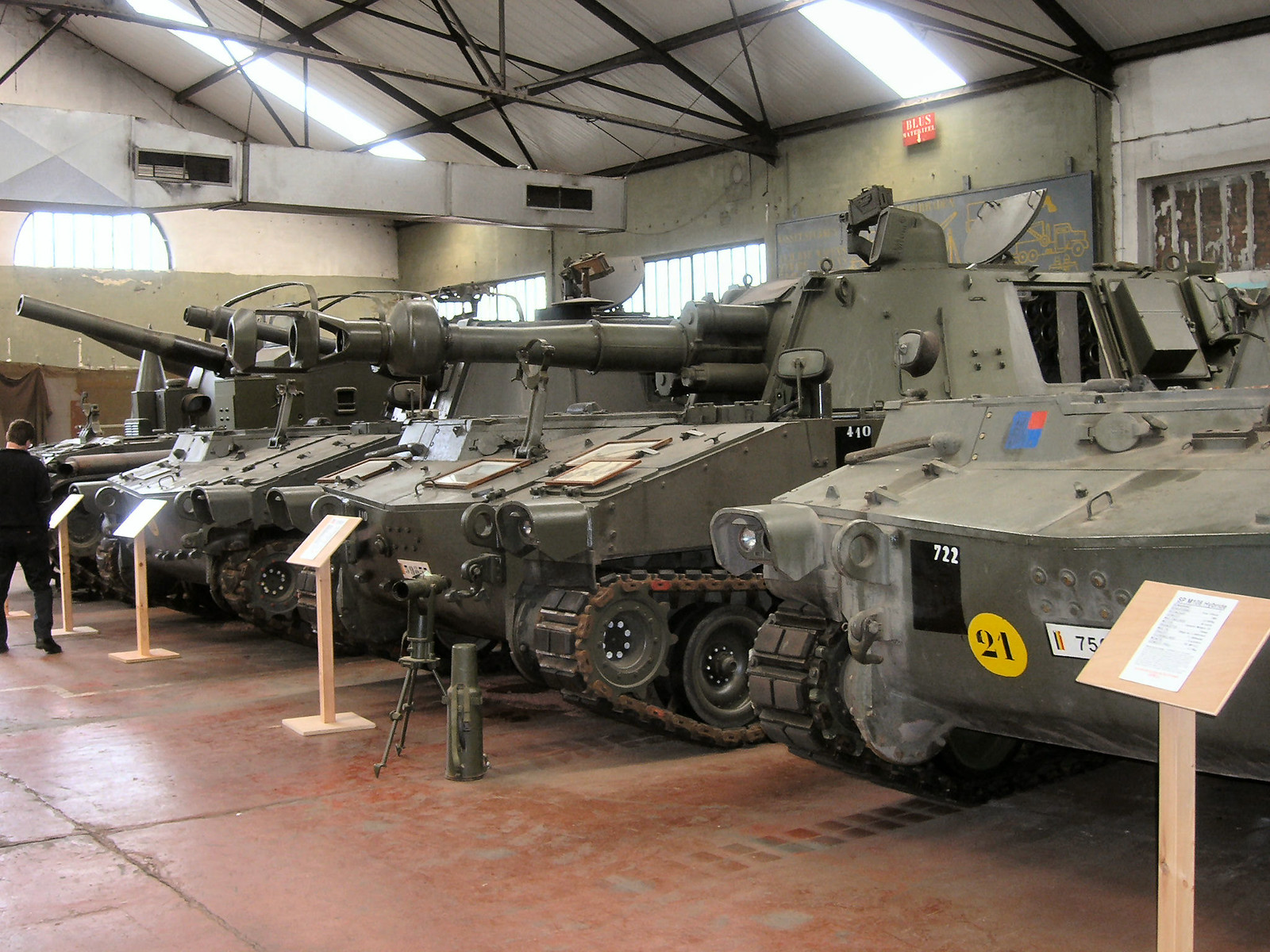The photograph depicts a landscape-oriented, color image taken inside a large, open metal hangar that has been converted into a museum housing various military tanks. The tanks, olive green in color, are arranged side by side in a row that stretches diagonally from the foreground on the right to the background on the left. Each tank is equipped with turrets pointing towards the front where they face wooden plinths. These plinths comprise a square base and an angled top with white papers displaying detailed information about each tank. The hangar's floor consists of very large, reddish tiles, almost one per tank, with dark brown join lines and some areas of damage. In front of one tank, there is even a mortar displayed. A Caucasian male dressed in all black is seen on the left side of the image, examining one of the plaques, while daylight streams in from the exterior, illuminating the scene.